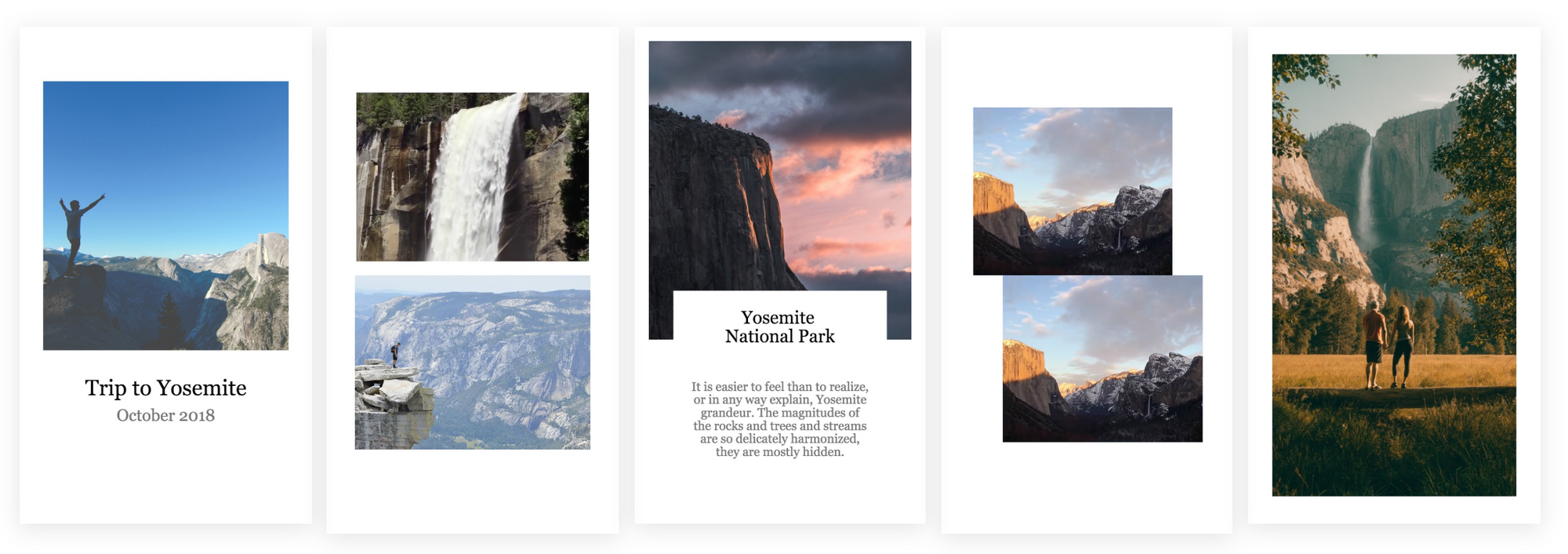Here is the refined and detailed caption:

"A series of five sets of images captures the breathtaking landscapes and memorable moments from a trip to Yosemite in October 2018. Arranged from left to right, the first set features a single picture of a person standing triumphantly atop a cliff, overlooking the rugged, mountainous expanse. The second set includes two images: the upper photograph showcases a majestic waterfall cascading down rocky terrain, while the lower image mirrors the first set, with another person standing at the edge of a cliff, surveying the vast scenery. The central set prominently displays the title 'Yosemite National Park' against the backdrop of a towering, steep cliff, accompanied by a descriptive paragraph beneath. In the middle-right set, two nearly identical images beautifully capture the interplay of shadows cast by the mountains. The final set on the far right depicts two individuals standing in an open field, gazing up in awe at a lofty waterfall in the distance. This visual narrative eloquently conveys the awe-inspiring natural beauty and adventurous spirit of Yosemite National Park."